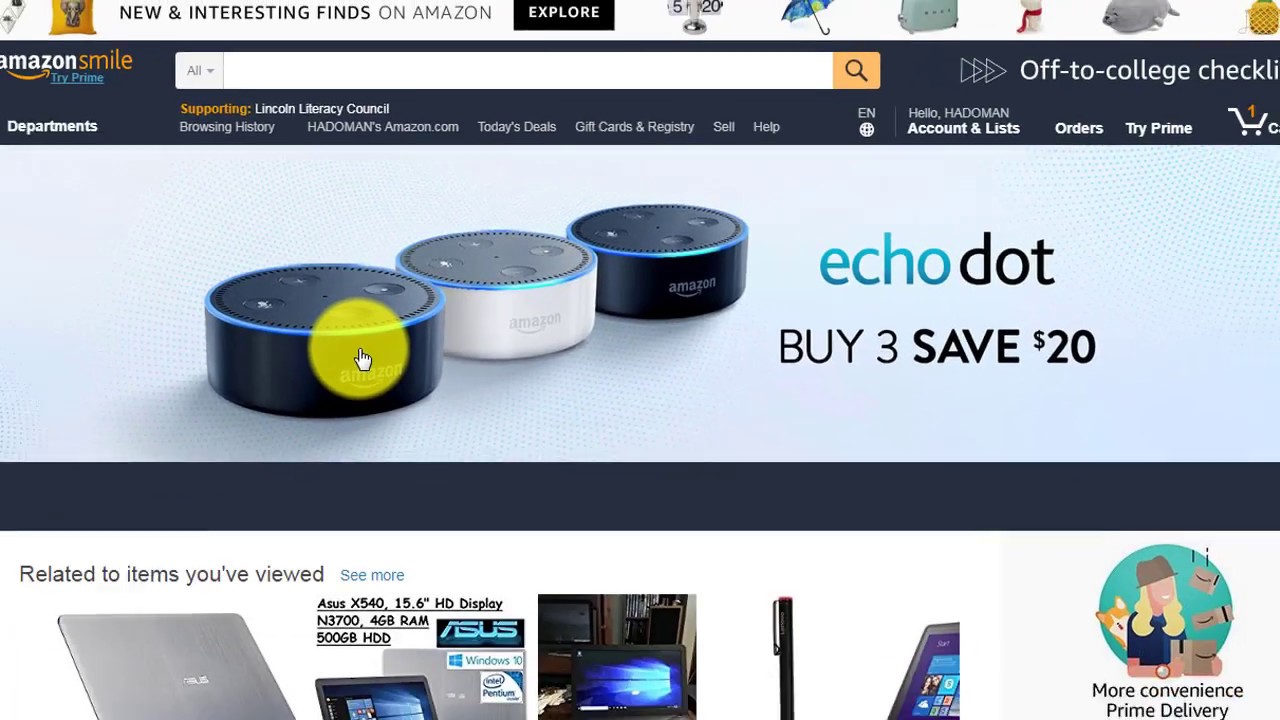The image depicts an Amazon Smile page with a prominent blue link encouraging users to "Try Prime" below the "Amazon Smile" logo. A search bar with a drop-down menu set to "All" and an orange search button labeled "Off to College Checklist" is positioned on the right. Below the search bar are various navigational menus including "Browsing History," "Hattoman's," "amazon.com," "Today's Deals," "Gift Cards & Registry," "Sell," and "Help." On the right side of the screen, the user's account section greets "Hello, Hattoman" and features options for "Accounts & Lists," "Orders," "Try Prime," and a cart indicating one item.

A large advertisement for Echo Dot dominates the midsection, showcasing three Echo Dots aligned diagonally facing the bottom right. The Echo Dots include a black one on either side and a white one in the middle, accompanied by the offer "Buy three, save $20."

Further down, a section titled "Related to items you've searched," features images of two Asus laptops, another Windows screen, and a pen, with a blue "See More" button for additional related items.